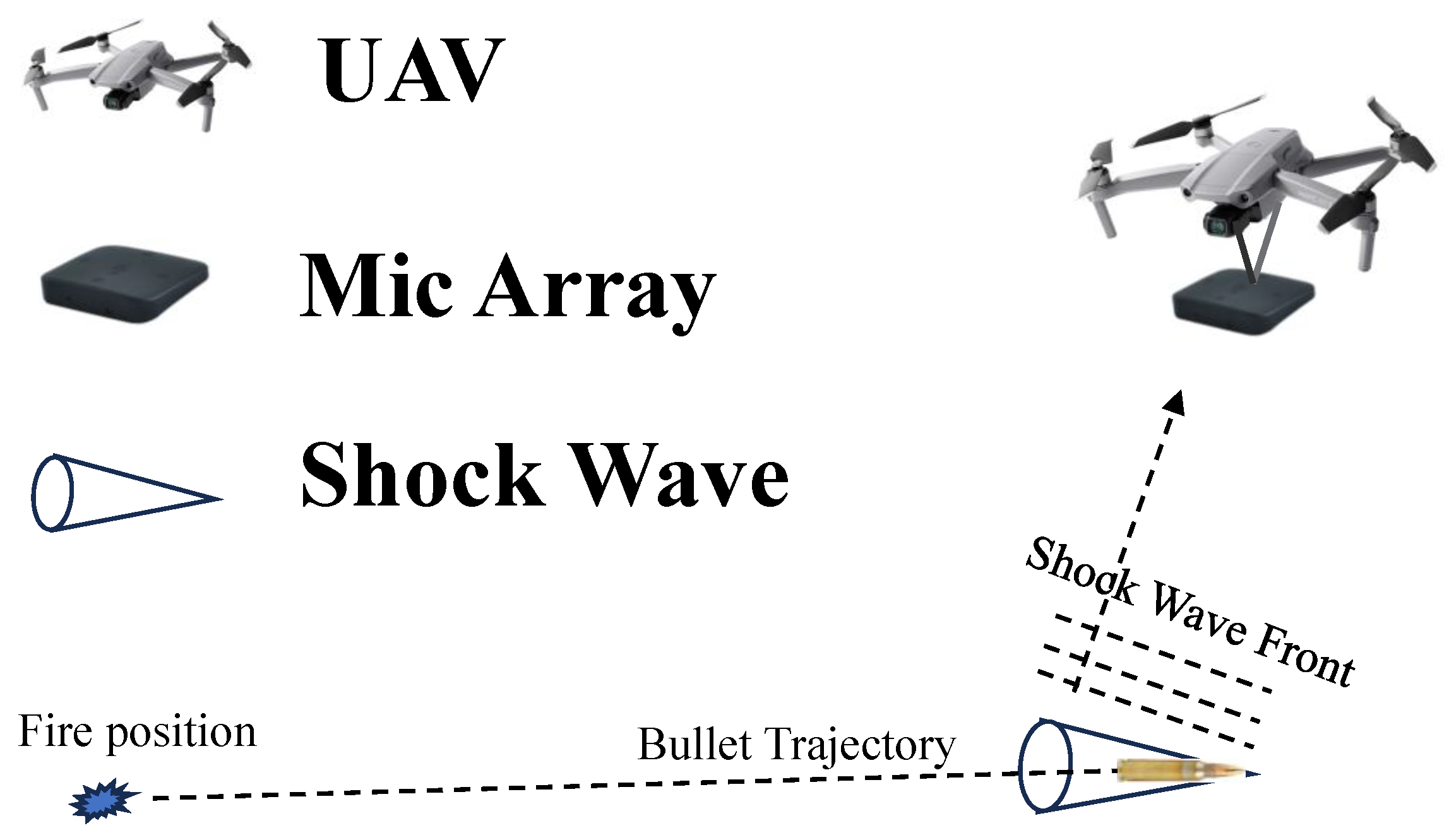This detailed image depicts a chart set against a white background, focusing on a sequence of components related to UAV operation. On the upper left, a gray drone labeled "UAV" is prominently depicted with four rotors extending outwards, two on each side. Hanging below the UAV is a black, cube-like object labeled "MIC array," resembling a small streaming device. Adjacent to these at the top, there is a cone-shaped diagram marked "shockwave."

Beneath these labeled elements, the chart unfolds starting at a point denoted "fire position," signified by a blue starburst. From this origin, a dotted line representing the "bullet trajectory" extends horizontally to the right, moving through the shockwave cone. The trajectory then angles upward, heading toward the UAV and the MIC array, which appears to act as the base for the shockwave cone. Additionally, the chart highlights the "shockwave front" with numerous dotted lines pointing up towards the drone and its attached MIC array.